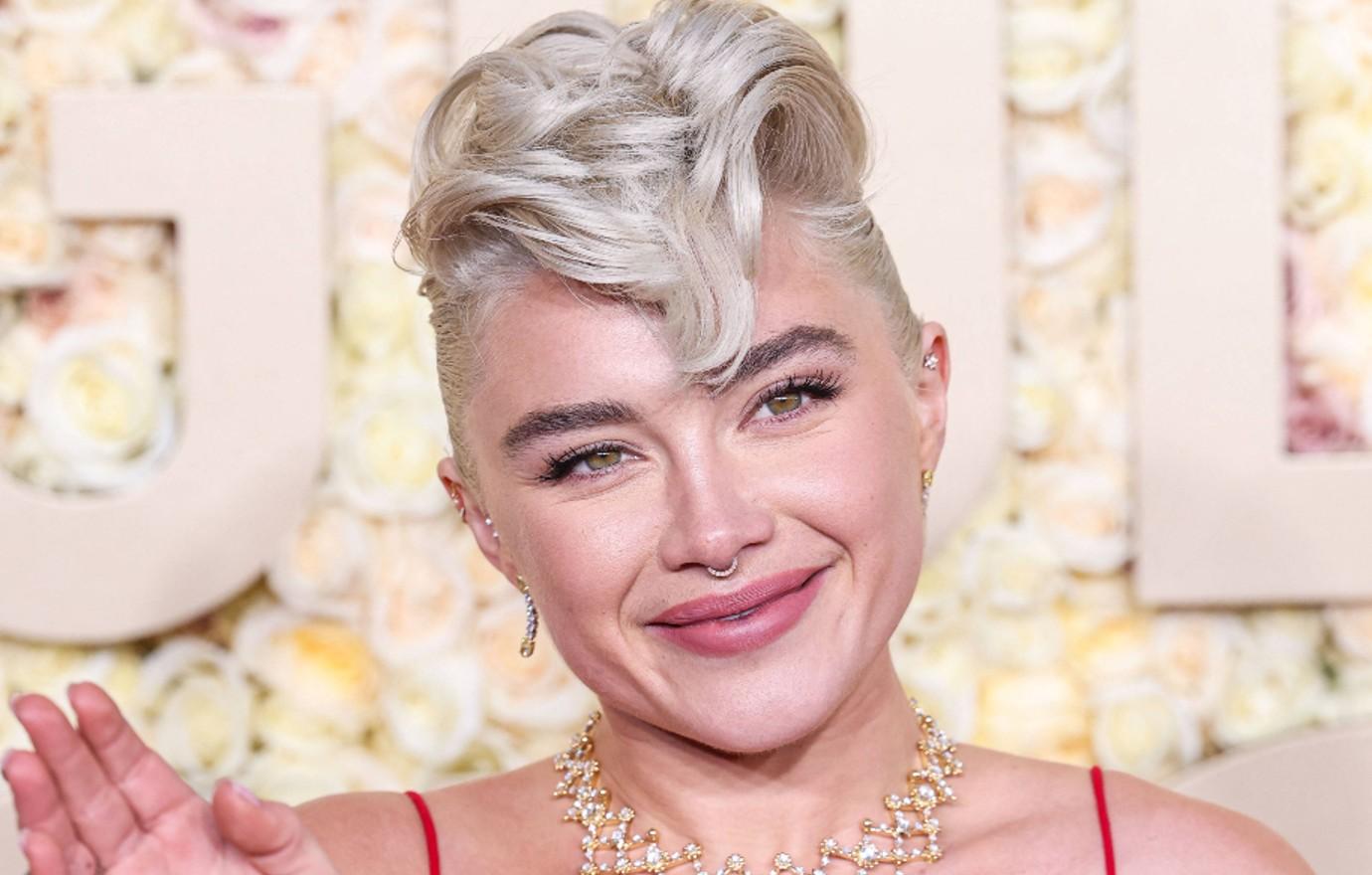This close-up photograph features an actress with a distinctive and unusual hairstyle. Her short, bleached blonde hair is tightly pulled back on the sides, with longer, curled sections that fall forward towards her eyebrows, emphasizing her thick, dark eyebrows. She has a playful smirk on her face, highlighted by red lip gloss. Her striking greenish-brown eyes appear slightly unfocused, with both eyes looking in different directions. Adorning her ears are multiple earrings, at least two per ear, varying in silver and gold. She sports a small, diamond-encrusted nose ring in her septum. Around her neck, she wears a snug, golden necklace embedded with diamonds, adding a touch of glamour to her look. She’s dressed in a red outfit, discernible by the thin red spaghetti straps over her shoulders. The rest of the dress isn’t visible, but the background includes a wall with cut-out letters that spell "Jill." She appears to be waving with her right hand, although the gesture is partially cut off in the photograph.